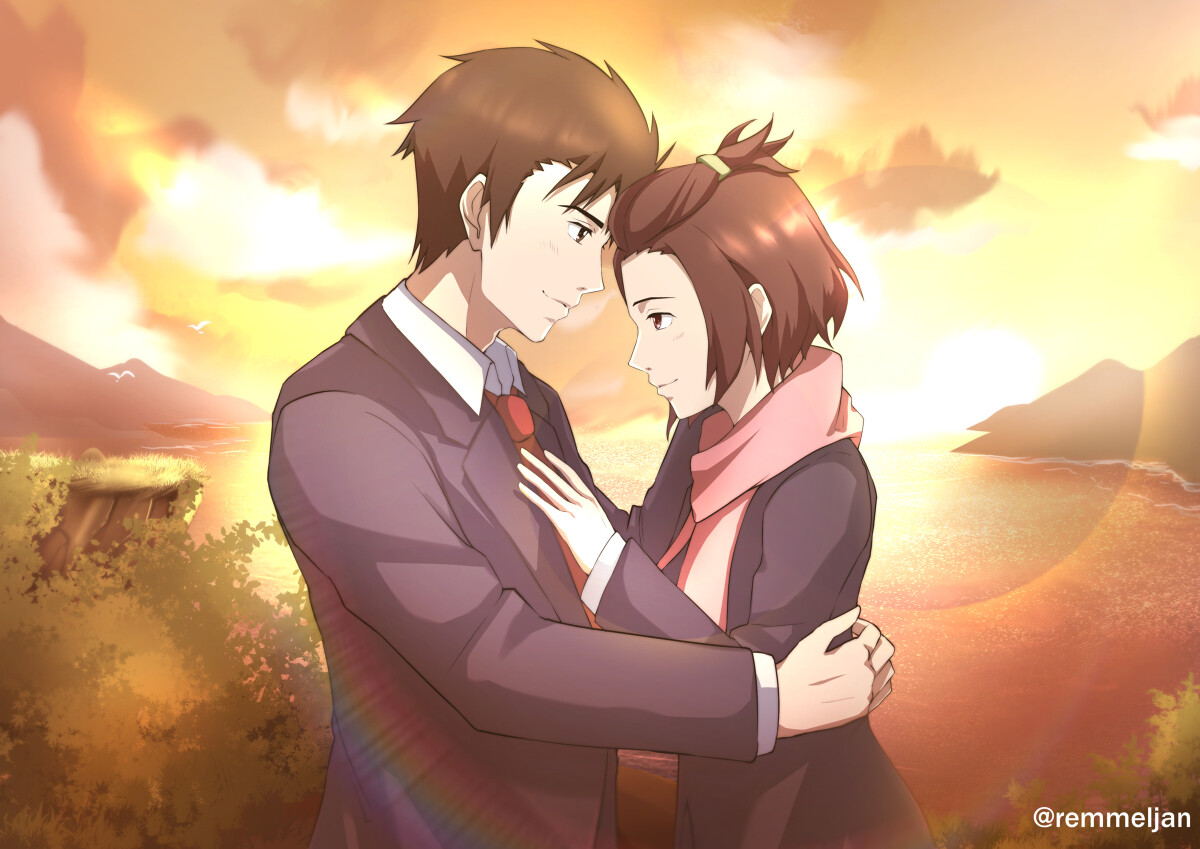In this captivating anime artwork, created by @remmeljan, we find a heartwarming scene set against a breathtaking sunset backdrop. The sky is ablaze with rich orangey and yellow tones, casting a warm, nostalgic glow over the serene hills and shimmering body of water in the distance. The composition also features lush foliage and leaves, adding a natural touch to the scenery.

At the forefront, a young couple stands close, deeply engrossed in each other's presence. The man, dressed in a suit with a red tie, gazes lovingly into the eyes of the woman, who wears a dark jacket and a delicate pink scarf. His arms are tenderly wrapped around her waist, while her hand rests gently on his chest, the other subtly adjusting his tie. Their brown hair captures the light of the setting sun, adding a touch of realism to the drawing. The woman’s short hair, partially clipped up with a yellow band, complements her serene demeanor.

Framing this touching moment is a circular rainbow and twinkling simulated lens flares that add a magical aura to the entire scene. The right side of the background reveals the sun sinking near the horizon, and the left side is dotted with bushes and grass, with a few seagulls soaring gracefully in the twilight sky. This detailed, lovingly crafted image is a beautiful representation of an intimate moment shared between two anime characters, making it a splendid piece of art.